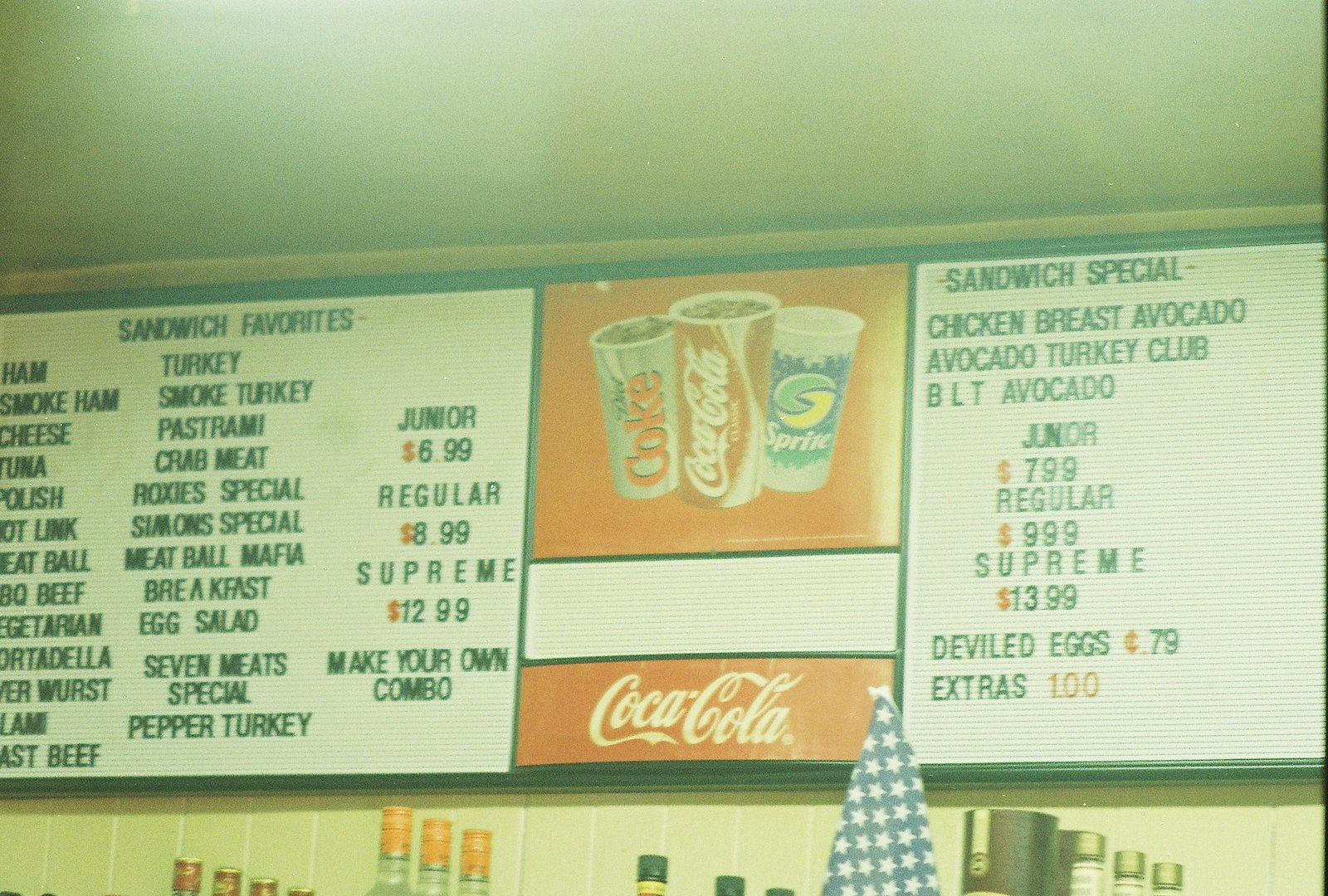The image depicts a restaurant's menu board mounted on a white-tiled wall. The board, framed in black, is predominantly white with black lettering and is divided into distinct sections. On the left side of the board, it features the heading "Sandwich Favorites" with listings such as ham, smoked ham, cheese, tuna, smoked turkey, pastrami, and crab meat, all accompanied by their respective prices.

In the center of the board, a red section highlights beverage offerings with images of Diet Coke, Coca-Cola, and Sprite cups. The Diet Coke cup is gray with red lettering, the Coca-Cola cup is red and white, and the Sprite cup is green and white.

To the left of this central section, the board displays another list under "Sandwich Specials," detailing options like chicken breast, avocado, avocado turkey club, and BLT avocado, along with their prices and available sizes. The ceiling above is white, and bottles are visible lined up along the tiled wall.